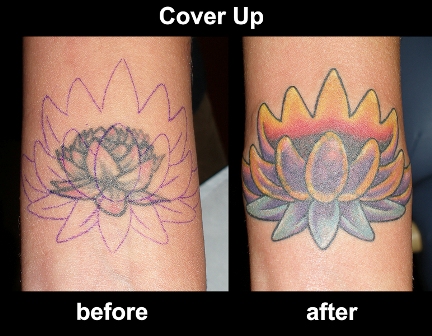This image is a detailed before-and-after comparison of a tattoo cover-up. Against a black background, the left side shows the "before" tattoo: a smaller design resembling a flowering cactus or succulent plant, accompanied by a blue outline indicating where the new tattoo will go. This original tattoo is not fully colored, displaying some scribbles and rough details in the center. Underneath, the word "before" appears in white text.

The right side displays the "after" image, featuring the completed tattoo that has fully covered the old one. This new design is significantly larger and more vibrant. It retains a cactus-like appearance but is thoroughly colored, with a yellow and red interior and bluish-green outer sections. Yellow highlights accentuate the exterior, while the leaves at the bottom exhibit a more pure blue-green hue. The arm sporting the new tattoo appears slightly skinnier than in the "before" image. At the top, the text "cover-up" is written in white, and beneath both photos, the words "before" and "after" are displayed.